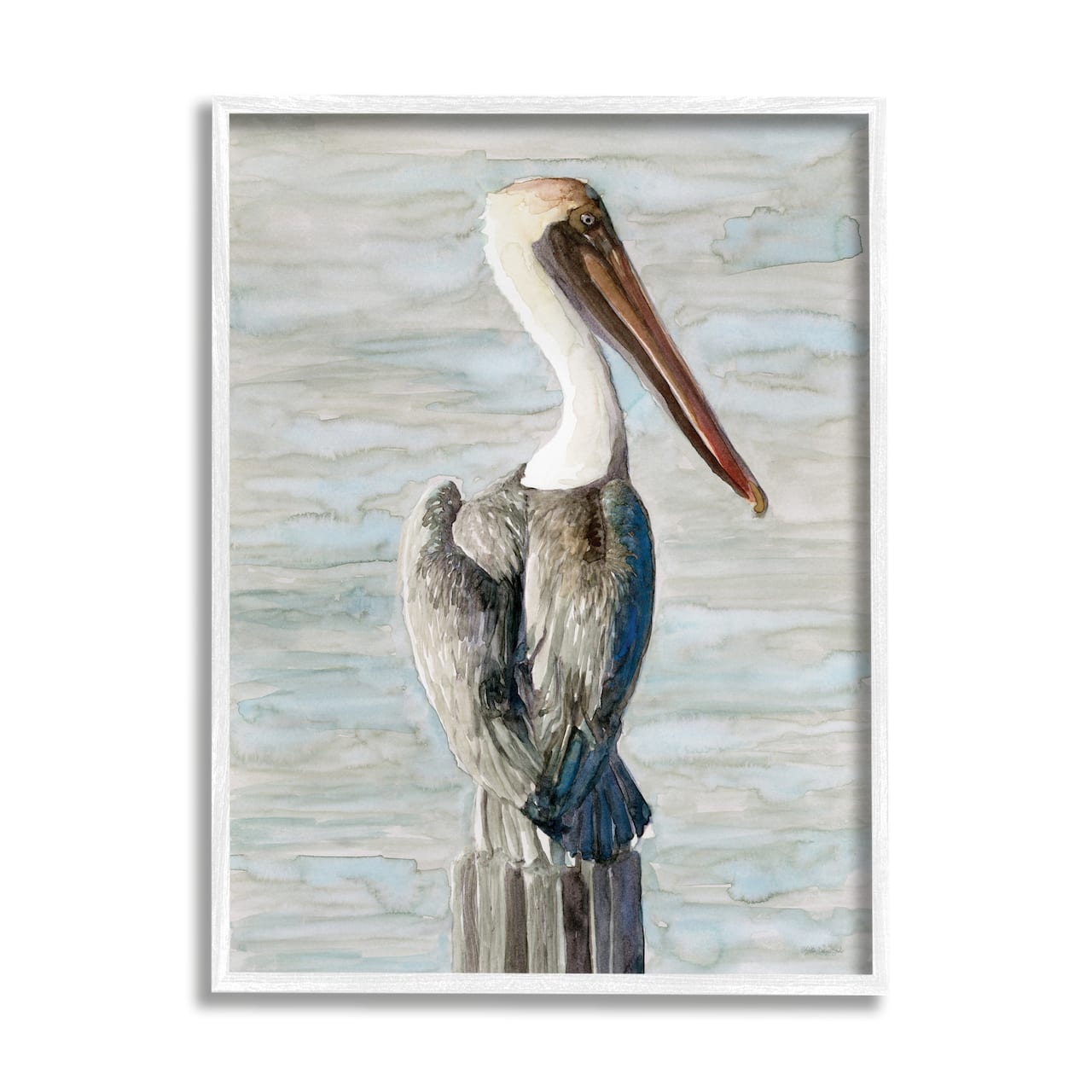This detailed depiction showcases a framed painting of a pelican, characterized by its distinctive and accurate portrayal through soft, light colors that suggest it might be done in watercolors. The background consists of a grayish, pale green, and bluish-gray palette, resembling gentle ocean waves. Central and prominent within the image, the pelican perches on top of a wooden post jutting out of the water, appearing restful with its folded wings closely held to its gray body. The feathers display varying shades of gray, with the rear wing feathers showing a bluish tint. The pelican's neck, stark white, transitions smoothly into a beige-tinted cap on its head, culminating in a long, diagonally-drooping brown beak that subtly curves into a yellowish tip. Notably, the bird's small, silver-ringed eye, black-centered, adds a striking detail to this calm, serene depiction of the seaside bird.